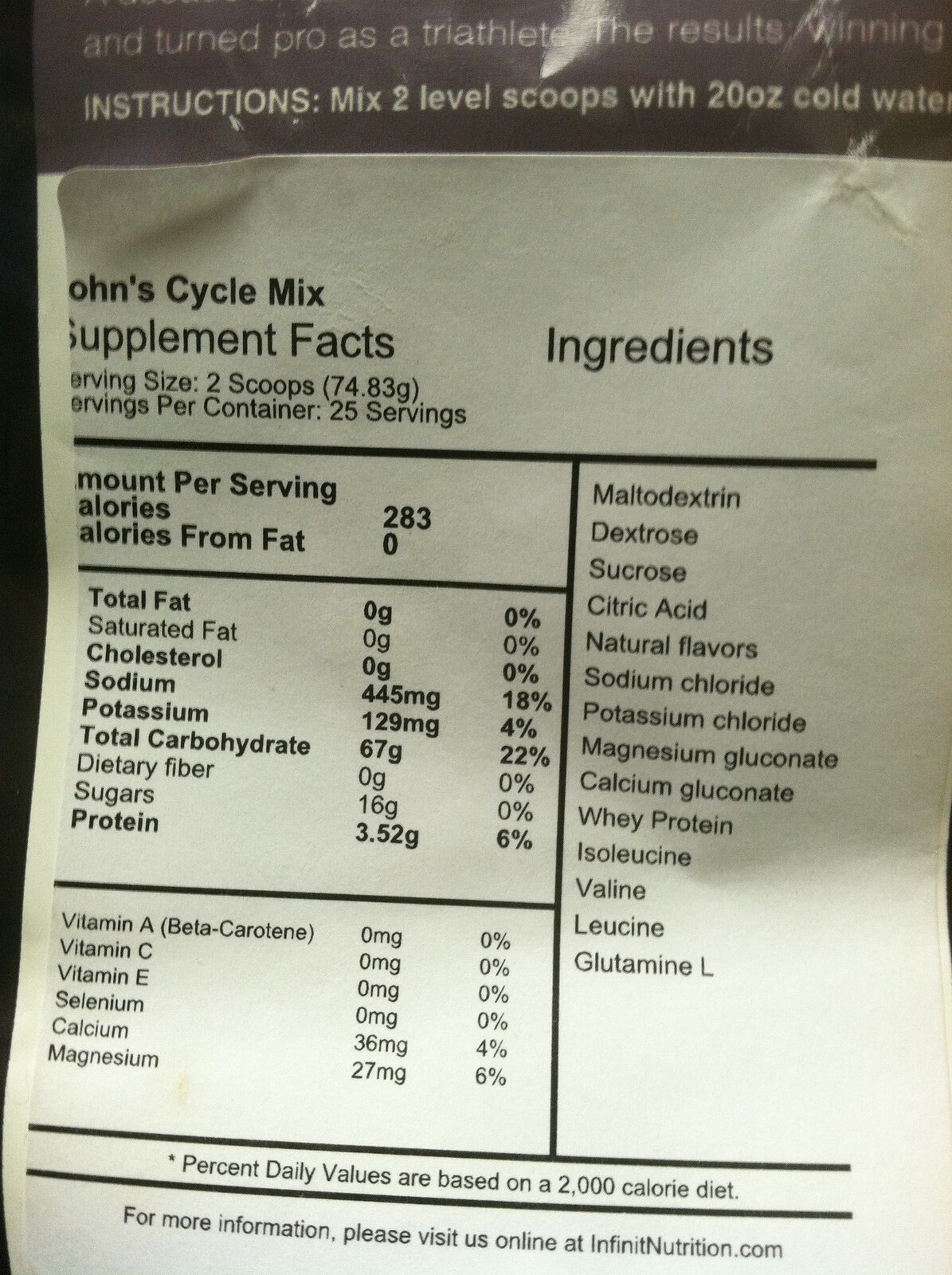The image is a color photograph of the back of a nutritional supplement package, specifically "John's Psycho-Mix." The package features a white paper-like label glued onto a purplish background. At the top, there are instructions in black ink that read: "Mix two level scoops with 20 oz cold water." Below the instructions, the label highlights "Supplement Facts," including details such as serving size (two scoops), servings per container (25 servings), and amounts per serving. The nutritional breakdown lists calories (283), calories from fat (0), total fat, saturated fat, cholesterol, sodium, potassium, total carbohydrates, dietary fiber, sugars, and protein. Additionally, it includes a comprehensive list of vitamins and minerals like Vitamin A, Vitamin C, Vitamin E, selenium, calcium, and magnesium. The ingredients, positioned on the right side, include maltodextrin, dextrose, sucrose, citric acid, calcium gluconate, protein, isoleucine, and valine. The bottom section of the label directs users to visit infinitynutrition.com for more information.